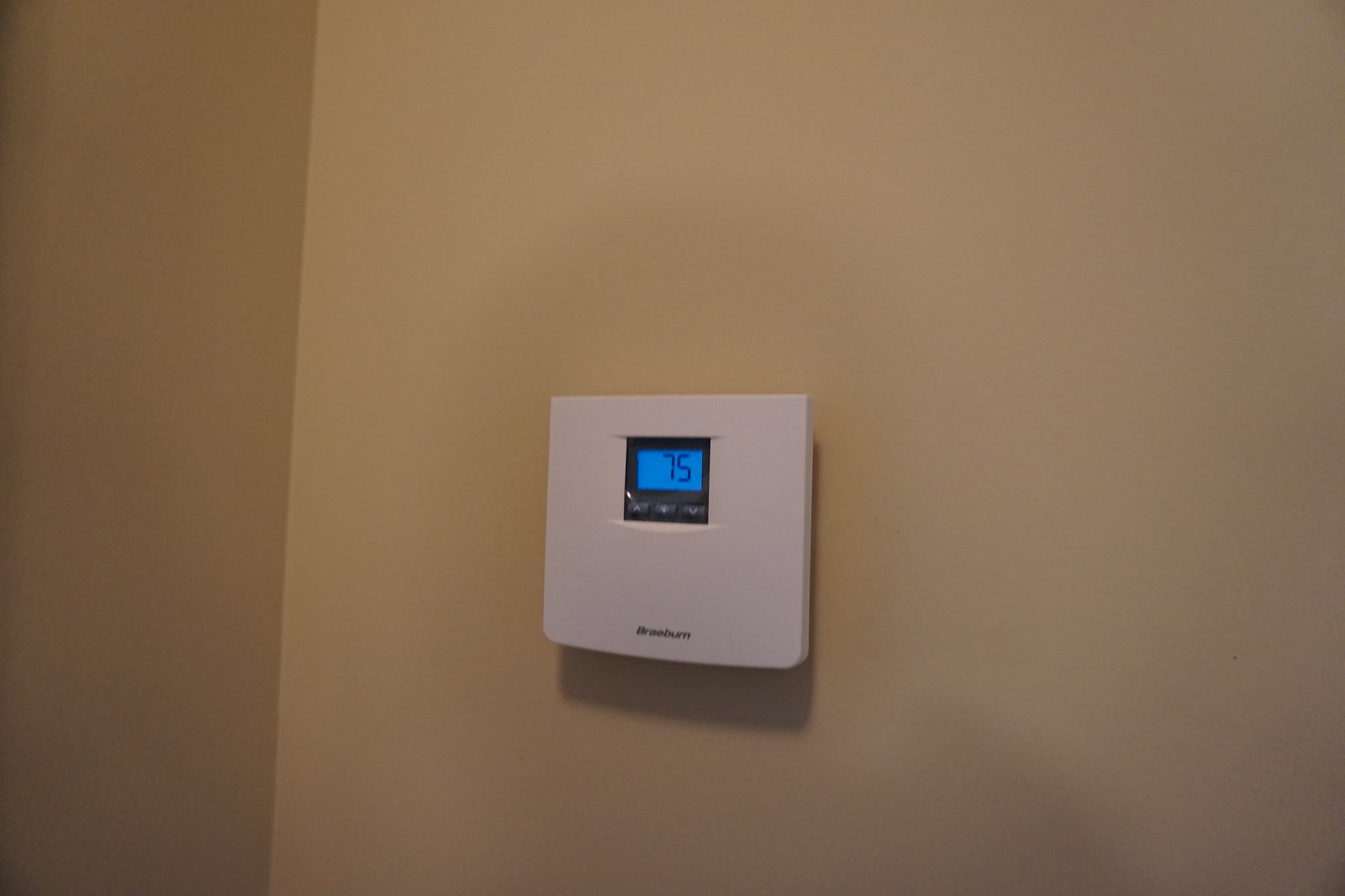The image depicts a cream-white corner wall featuring a mounted digital thermostat. The thermostat, primarily white, includes a blue screen that prominently displays the number "75," indicating the current room temperature in Fahrenheit. The device has several buttons and a black outline around the screen. Positioned slightly off-center, the thermostat bears some unreadable brand-related text at its bottom, printed in black. The perspective of the photograph is from a frontal angle, capturing the thermostat within a corner setting.